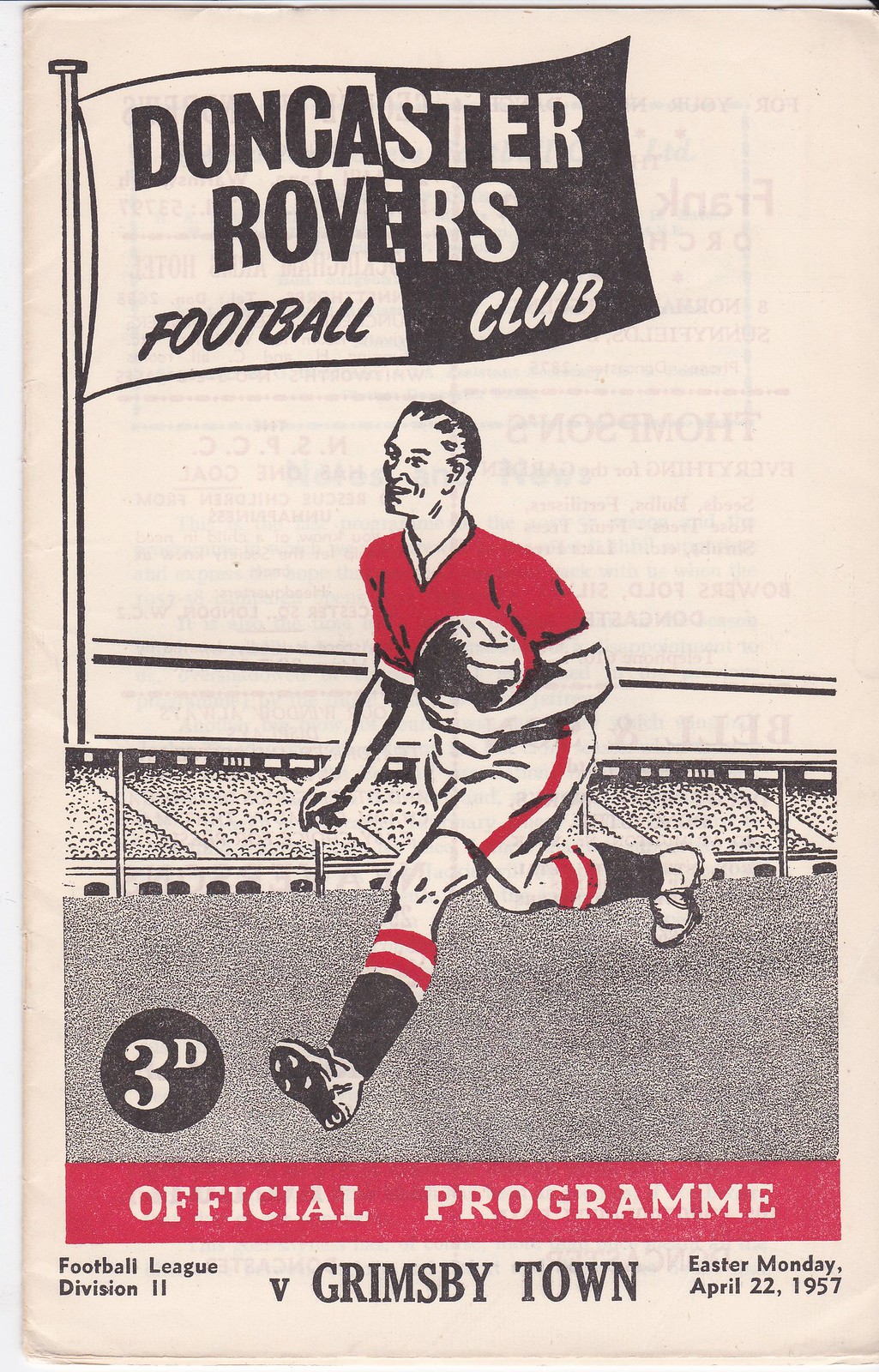This image depicts the vintage cover of an official matchday program for Doncaster Rovers Football Club. The background of the cover has a paper-colored tone, typical of the era. In the top left corner, there is an illustration of a flag, divided vertically; the left side is white with black text, and the right side is black with white text, collectively reading "Doncaster Rovers Football Club."

Beneath the flag, a detailed cartoon of a footballer is featured. The player is depicted running with a soccer ball, even though in actual gameplay, a player would not carry the ball unless he is the goalkeeper, which this character does not appear to be. The footballer is dressed in a red jersey, white shorts with a red stripe down the side, and white socks with two red bands at the top and black at the bottom. He is portrayed running on a stylized pitch with an outlined drawing of stadium stands behind him, filled with tiny circles representing the crowd. A flag emerges from these stands, further adding to the scene's lively atmosphere.

At the bottom of the cover, a red banner features the words "Official Programme" in white text. Information about the match appears below this banner: "Football League Division 2 vs. Grimsby Town" on the left, and "Easter Monday, April 22, 1957" on the right. Additionally, the price "3d" is indicated within a black circle with white text. The hints of another newspaper article can faintly be seen in the background, suggesting this program's print on characteristic thin paper.